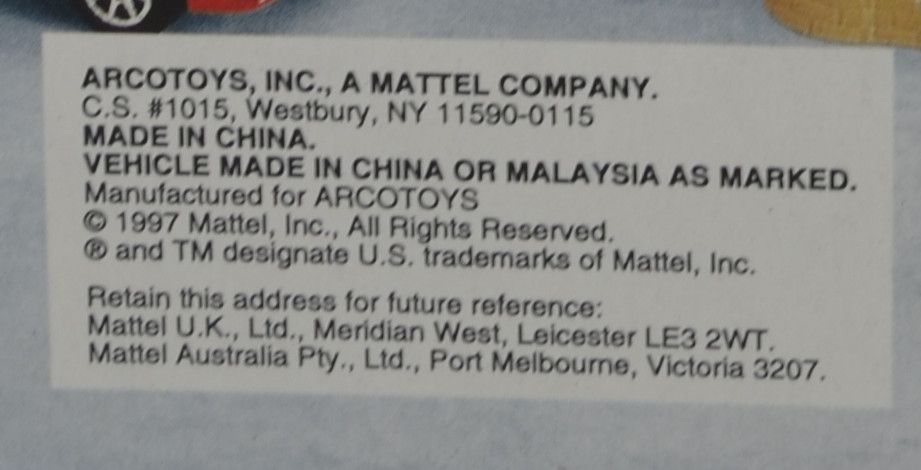This image displays a label for a toy vehicle manufactured by Arco Toys, a subsidiary of Mattel. The top left corner shows partial visuals of a tire and a red section of a car, providing a hint of the toy's design. In the top right corner, there is an unclear yellow brick-like object. The main portion of the label features the company name, "Arco Toys Incorporated, a Mattel company," and mentions its manufacturing origins in China and Malaysia. The label also lists multiple contact addresses for Mattel, including locations in New York, the United Kingdom, and Australia. Additionally, it indicates that the toy was made in 1997, with relevant copyright and trademark information.